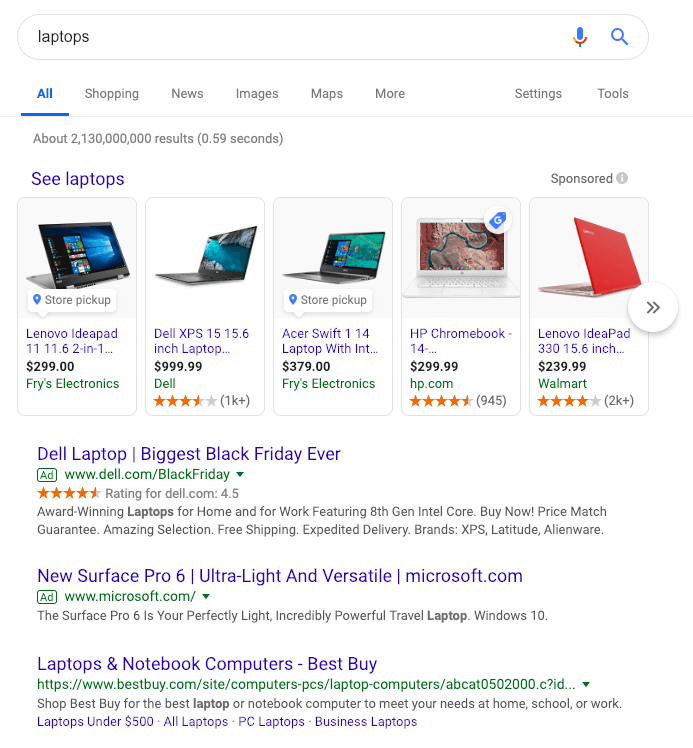The image is a screenshot of a Google search results page. The search query "laptops" is typed into the search bar at the top. Directly below the search bar, the Google tabs for "All," "Shopping," "News," "Images," "Maps," "More," "Settings," and "Tools" are visible, with the "All" tab selected. The search returned approximately 2,130,000,000 results in 0.59 seconds.

Immediately below, there is a prompt reading "See laptops," followed by a row of five sponsored ads featuring various laptops. The first ad showcases a Lenovo IdeaPad priced at $299, available from Fry's Electronics. The second ad features a Dell XPS priced at $999. The third ad is for an Acer Swift 1.14 laptop priced at $379, also from Fry's Electronics. The fourth ad displays an HP Chromebook priced at $299, available directly from HP.com. The fifth and final ad in this row presents a red Lenovo IdeaPad 330 with a 15.6-inch screen, priced at $239, available from Walmart.

Below these sponsored ads are regular search result listings. The first listing is another ad titled "Dell Laptop Biggest Black Friday Ever," linking to Dell.com/BlackFriday. The second listing is an ad for the "New Surface Pro 6," described as ultralight and versatile, linking to Microsoft.com. The third listing is not an ad but a standard search result titled "Laptops and Notebook Computers," linking to BestBuy.com.